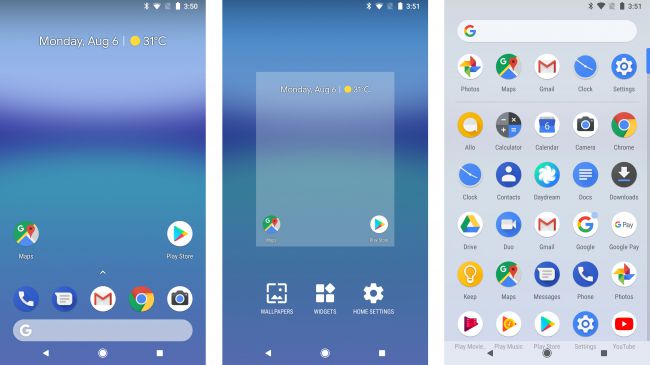A series of three sequential images showcasing the interface of a cell phone, likely the same device, as indicated by the consistent sequence of four icons in the upper right-hand corner and identical time stamps. The left image, captured at 3:50, displays a simple blue gradient background. The middle image at 3:51 shows the same blue gradient, now overlaid with a light gray or off-white screen selection in the center. The right image, also at 3:51, presents a list of applications against a solid gray background. The progression suggests that the user is navigating through their phone's settings, experimenting with different background screens within a short time span.